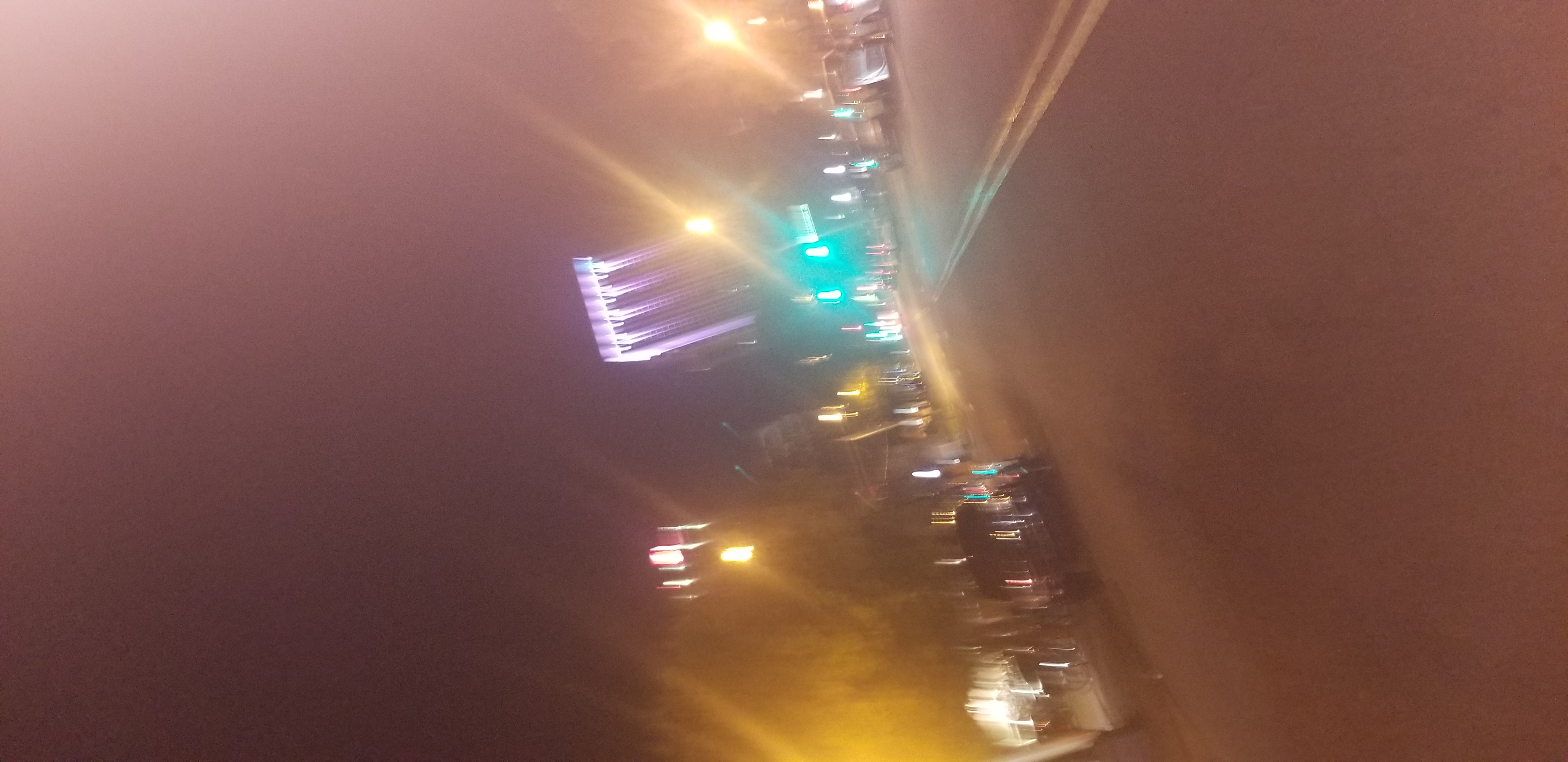A nighttime street scene captured with a hazy, dream-like quality. The photo, taken at an angle and appearing sideways, reveals a blurry dual lane road. Green traffic lights are visible in the distance, casting an eerie glow in the smoky air. Cars line both sides of the road, their shapes indistinct due to the blurriness. Ahead, five illuminated pillars punctuate the scene, accompanied by three street lights whose beams radiate outward, further enhancing the ethereal atmosphere.